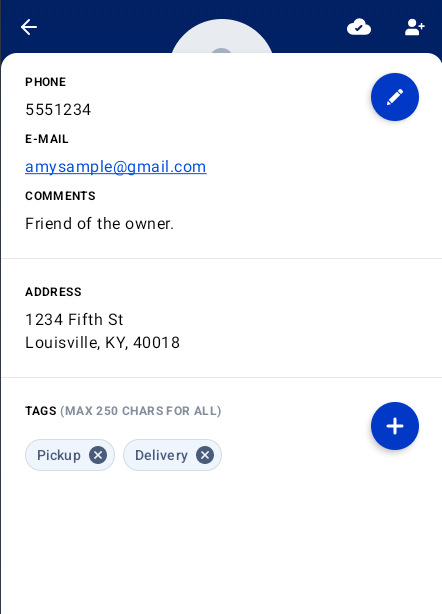The image is a screenshot displaying a structured interface on a cell phone, contained within a white rectangle with a blue border at the top. At the top left, a white arrow points to the left, indicative of a back navigation button. Below the arrow, a partially visible dome-shaped gray semicircle is cut off by the white background, while a white cloud icon with a black checkmark sits beside it.

At the top right, a person symbol with a plus sign suggests an option to add a contact. Directly below this symbol, the text "Phone: 555-1234" and "Email: anysample@gmail.com" are underlined in blue, denoting clickable hyperlinks that would allow users to directly call the phone number or compose an email.

Beneath this section, the text "Comments of friends of owner" appears followed by a light gray horizontal line. Under the line, the address "1234 5th Street, Louisville, Kentucky 40018" is listed, separated by another horizontal gray line below it. Further down, the text "Tags (max 250 characters for all)" appears, indicating a field for metadata, followed by two light blue tabs labeled "Pickup" and "Delivery."

A blue edit icon with a pencil inside is positioned to the far right of the phone and email information, suggesting the option to modify these details. In the Tags section, a blue circle with a white plus sign on the far right suggests adding new tags. This screenshot appears to be a template or example, as evidenced by the use of generic contact information and absence of additional text.